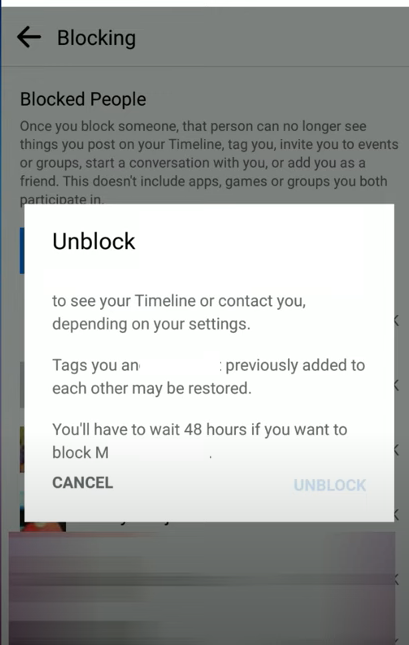The image depicts a user interface screen, likely from a social media platform such as Twitter or Instagram, focused on the blocking and unblocking features. In the center of the image, a large white dialog box appears with the title "Unblock" at the top. This dialog box contains instructions explaining that you will need to wait 48 hours to block someone again after unblocking them. The text also mentions restoration of previously added tags and connections once unblocked, although parts of this information appear erased or obscured. At the bottom of the dialog box are two buttons: one labeled "Cancel" in all caps, which is clearly visible and clickable, and another labeled "Unblock" on the far right, which is faded out and currently non-functional.

In the background, the top left corner features an arrow pointing to the left, labeled "Blocking." Below that, there is a section titled "Block People" with a brief description stating that once you block someone, they can no longer see your posts on your timeline, tag you, etc. This description is partially cut off and continues with "blah blah." A blue vertical sliver and some small boxes, presumably user profile pictures, are visible to the left of the white dialog box. There are about four different profile pictures partially shown underneath the dialog box, indicating other users on the platform.